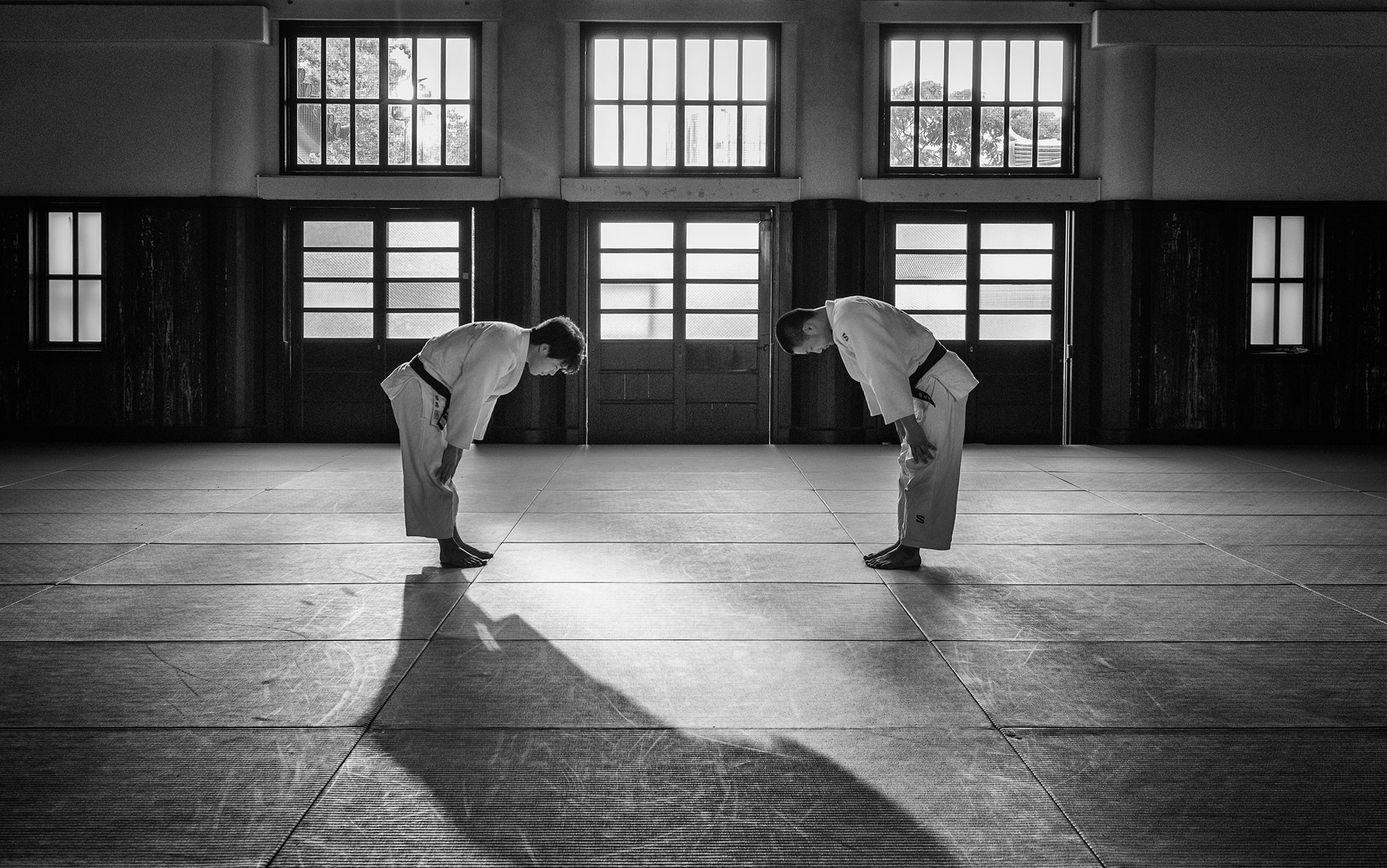This black and white photograph captures a serene moment in an otherwise empty karate studio, where two Asian men, each wearing a traditional karate uniform and a black belt, are bowing toward each other in a display of mutual respect before what appears to be a sparring session. Both men, who have dark, short hair, are leaning forward with their hands placed on their knees or thighs, reflecting a disciplined posture. 

In the background, the studio is illuminated by the light streaming through eight windows. These windows are arranged with two individual ones framing the scene on the far left and far right, while in the center, there are three stacks of double-paned windows. The detailed clarity of the shadows on the wooden or paneled floor adds to the image's aesthetic depth, creating a quiet yet anticipatory atmosphere as we sense the calm before the action begins. The composition of the photo, combined with the traditional dojo elements and the overlay of shadows, evokes a timeless and respectful spirit of martial arts practice.